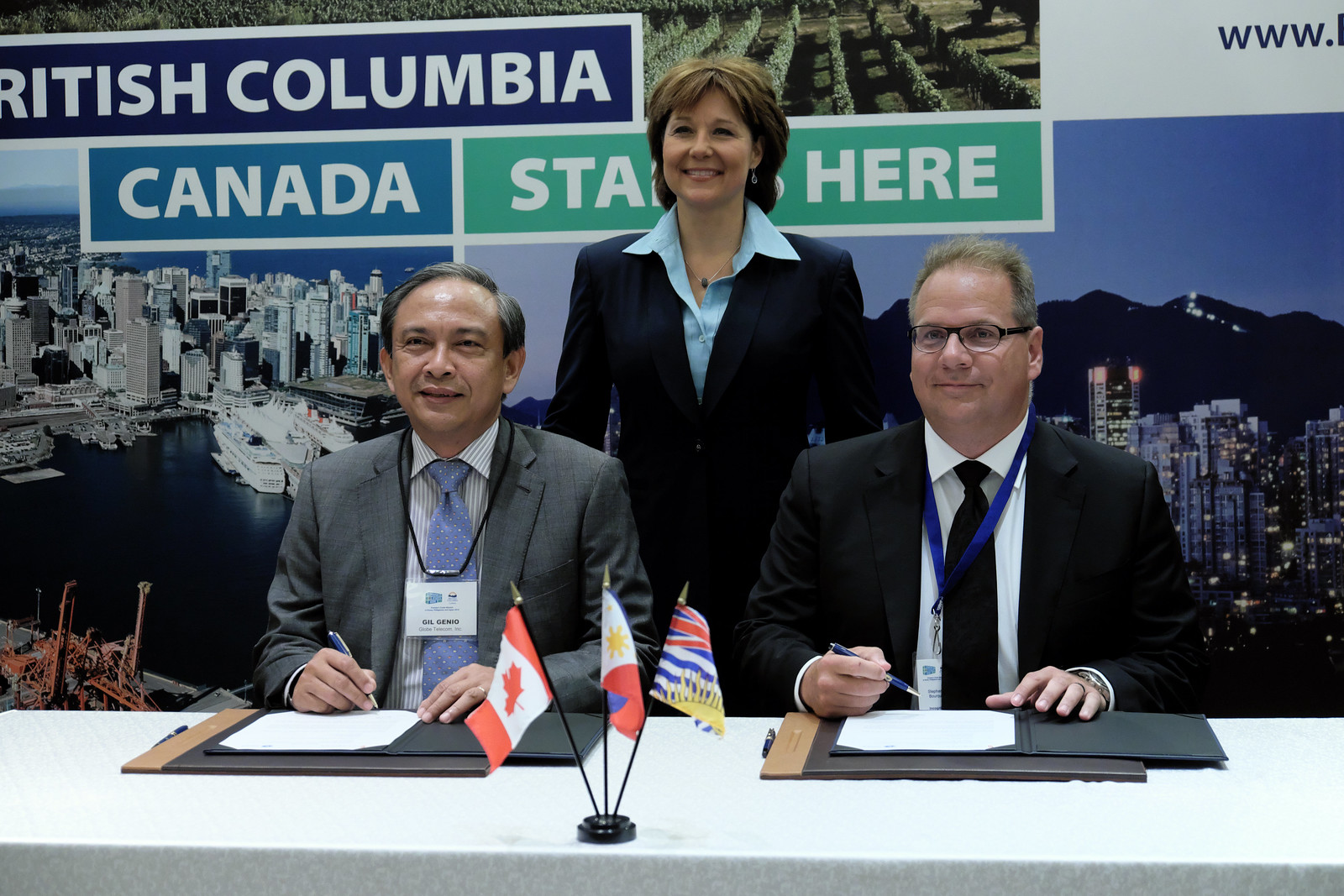In the photograph, two men are seated behind a white table covered with a white tablecloth, featuring a tiny black puck and three small flagpoles displaying the Canadian flag and two more local flags, possibly including a New Zealand flag. A woman stands between them, wearing a dark blue blazer over a light teal open-collar shirt. Behind them is a promotional board with images of a city, a city at night, and a farml field, overlaid with white text reading "British Columbia Canada starts here."

The man seated on the left is signing a piece of paper in a black folder. He is dressed in a gray suit, a light purple tie, and a gray and white striped button-up shirt, with a blue lanyard and an ID tag around his neck. The man on the right is wearing a black suit with a black tie, a white button-up shirt, and also has a blue lanyard with an ID tag.